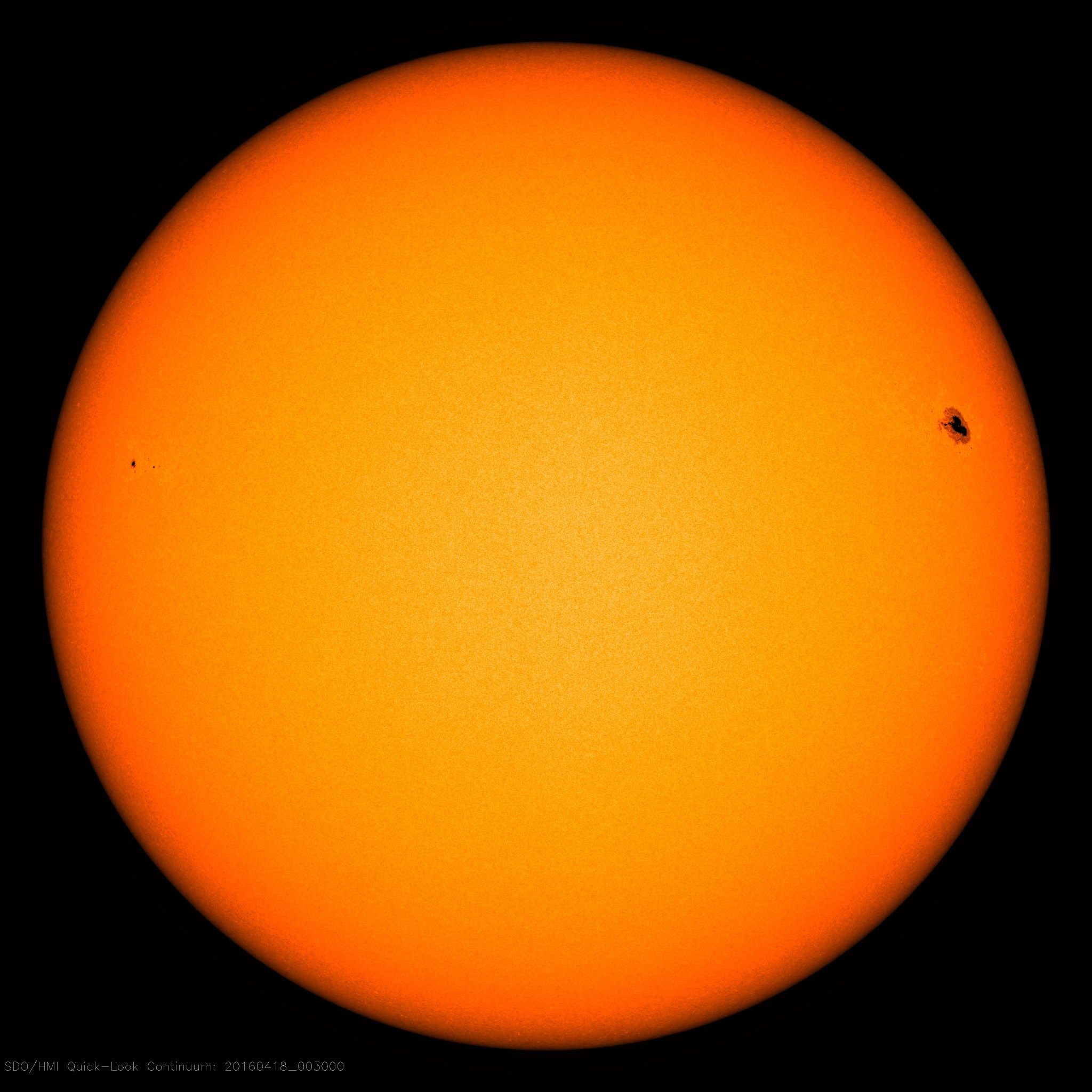This is a detailed, square image centered on a glowing, amber-colored orb against a jet black background. The orb has a vibrant fiery orange perimeter, which gradually transitions into shades of lighter orange before culminating in a radiant yellow at the center. The orb’s edges appear slightly blurred, suggesting it might be a distant object, possibly a planetary body or a light source like the sun or a light globe. Upon closer inspection, a small black blemish is noticeable on the far right side of the orb, resembling the outline of a common housefly, as if it's embedded within the glowing surface. This adds a peculiar, almost enigmatic detail to the image.